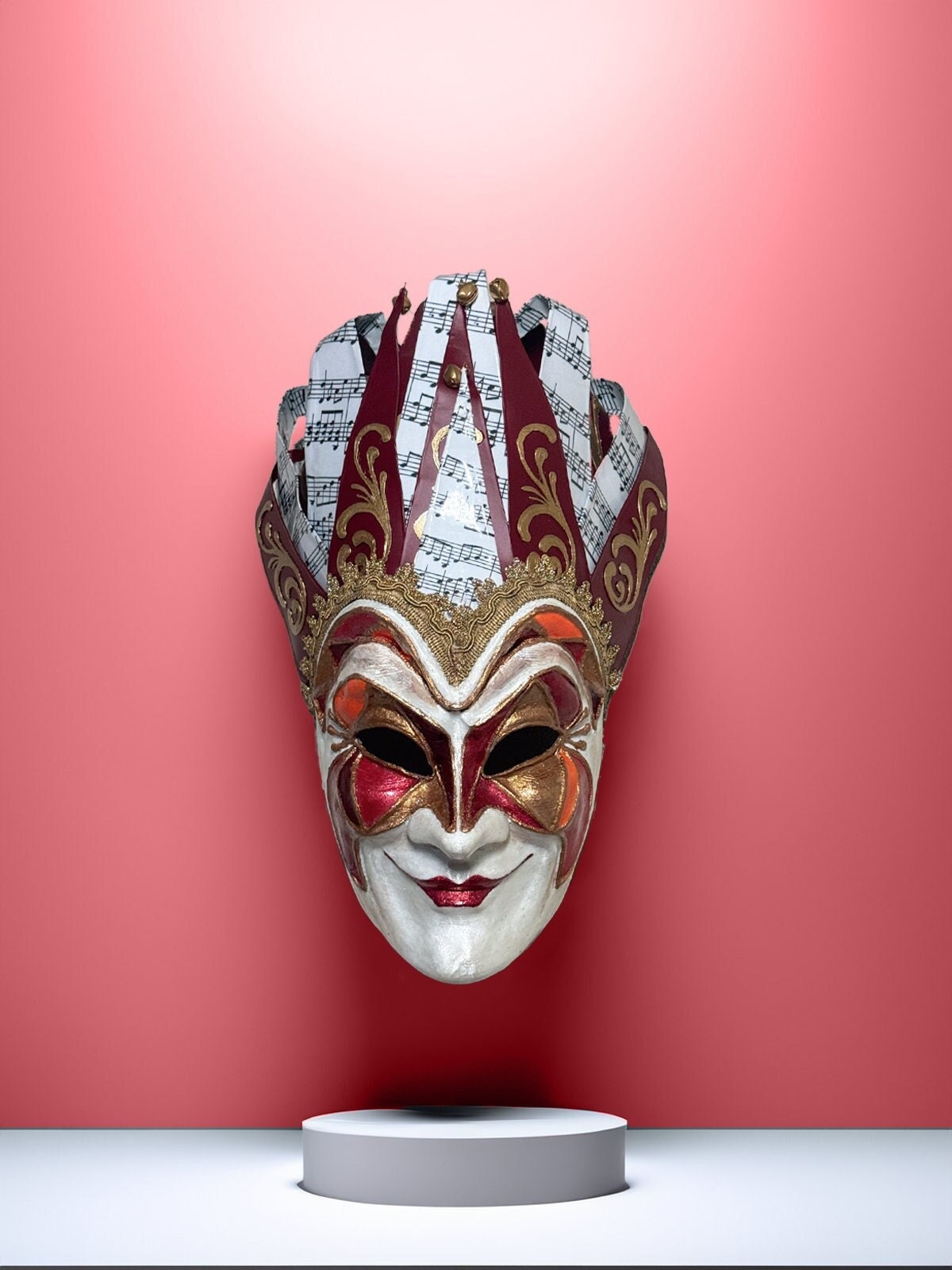The photo captures an elaborate mask displayed prominently against a bright, pinkish-red background. The mask, which is mounted above a short, white cylinder on a solid white surface, evokes the intricate designs often seen in costume parties and music festivals. This particular mask, reminiscent of those worn by techno artist Boris Breka, features a white face with striking, upturned dark red lips, mimicking a broad smile. The eye areas are adorned with a butterfly-shaped pattern in shades of red and gold. Atop the mask sits an elaborate crown-like adornment, with some segments showcasing dark red and gold swirls, while other segments display musical notes printed on a white background, adding to the mystique and artistic flair of the piece. The mask is illuminated from above, enhancing its vivid and ornate details.